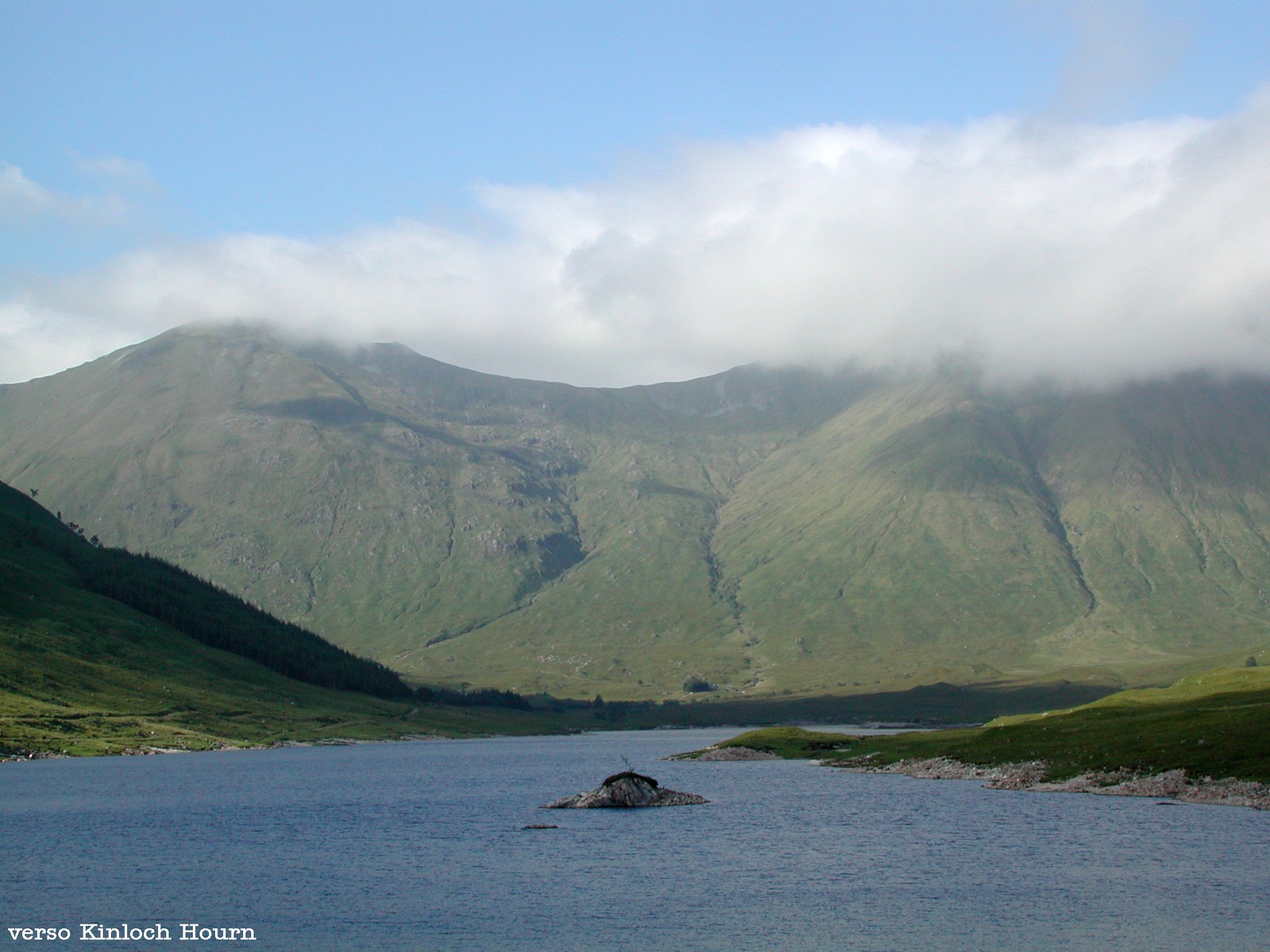This full-color aerial photograph, taken by Kinloch Horn, captures a breathtaking mountain range during the daytime. The mountains are lush and green, with their tall texture accentuated by low-hanging, fluffy white clouds and a clear blue sky above. Below, a large body of blue water with visible ripples stretches out, flanked by grassy fields on either side. On the left shore, a patch of grass and a small rock formation resembling a tiny island can be seen. The right side features steep grassy fields. The overall scene exudes natural beauty, framed by shadows and overcast light, lending it a serene and pristine atmosphere. The bottom left corner is inscribed with "Verso, Kinloch Horn," identifying the photographer and location.